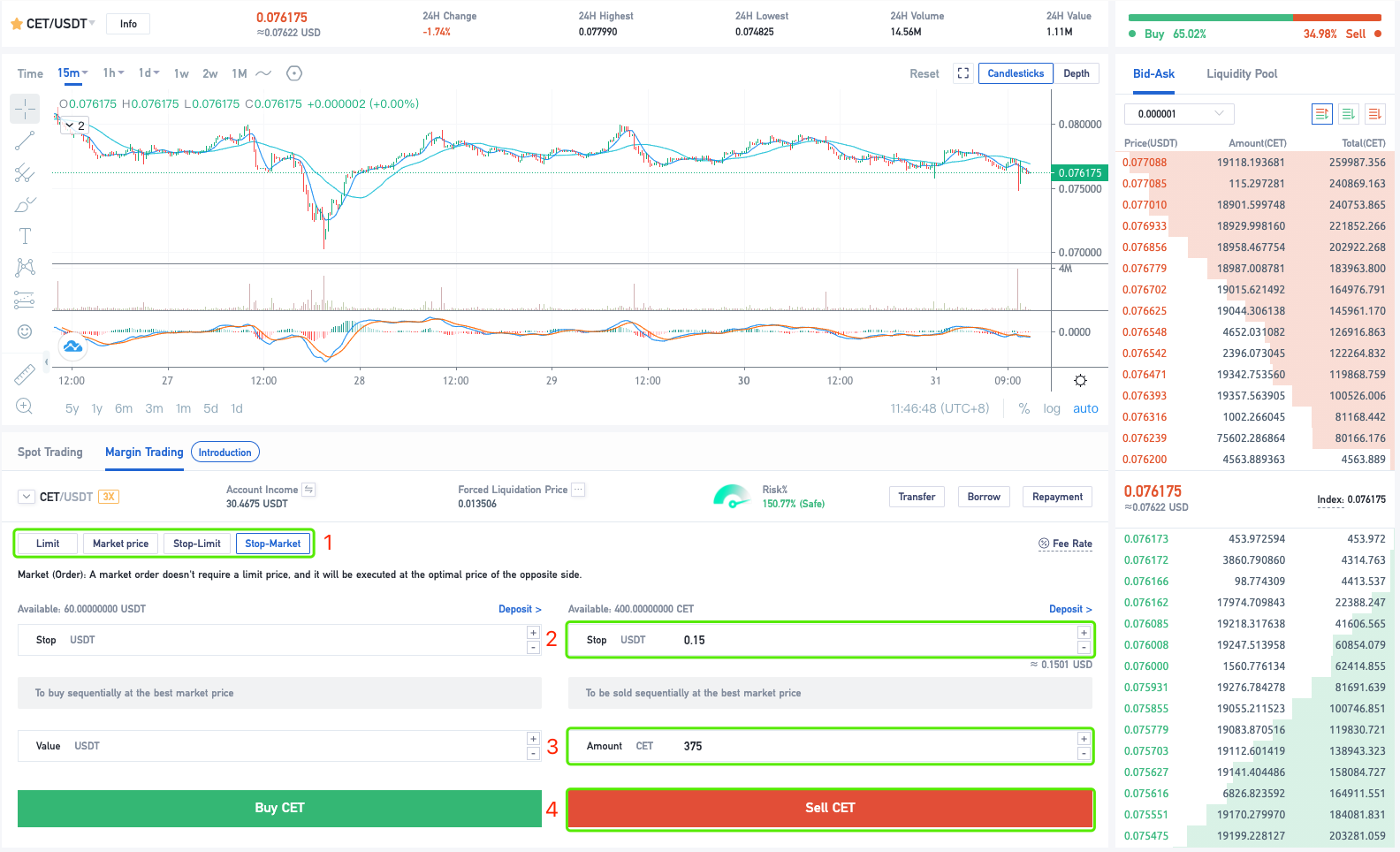In this image, a cryptocurrency trading dashboard is displayed, focusing on the CET (CoinEx Token) against USDT (Tether). The current value of CET is shown as 0.076175 USD, approximately 0.07622 USD, with a 24-hour change of -1.74%. The dashboard includes various features for traders, such as sports trading, margin trading, and account management tools. The account income is highlighted as 30.4675 USDT with a forced liquidation price set at 0.013506 USD. Traders can see different order types including limits, market price, and stock market orders. The market order feature is underscored, explaining that it will be executed at the optimal price of the opposite side without requiring a limit price. Additionally, there is information on available funds, specifying 60 USDT available for trading CET at the best market price. The value of CET in USDT is featured prominently, providing traders with clear options to buy CET using USDT.